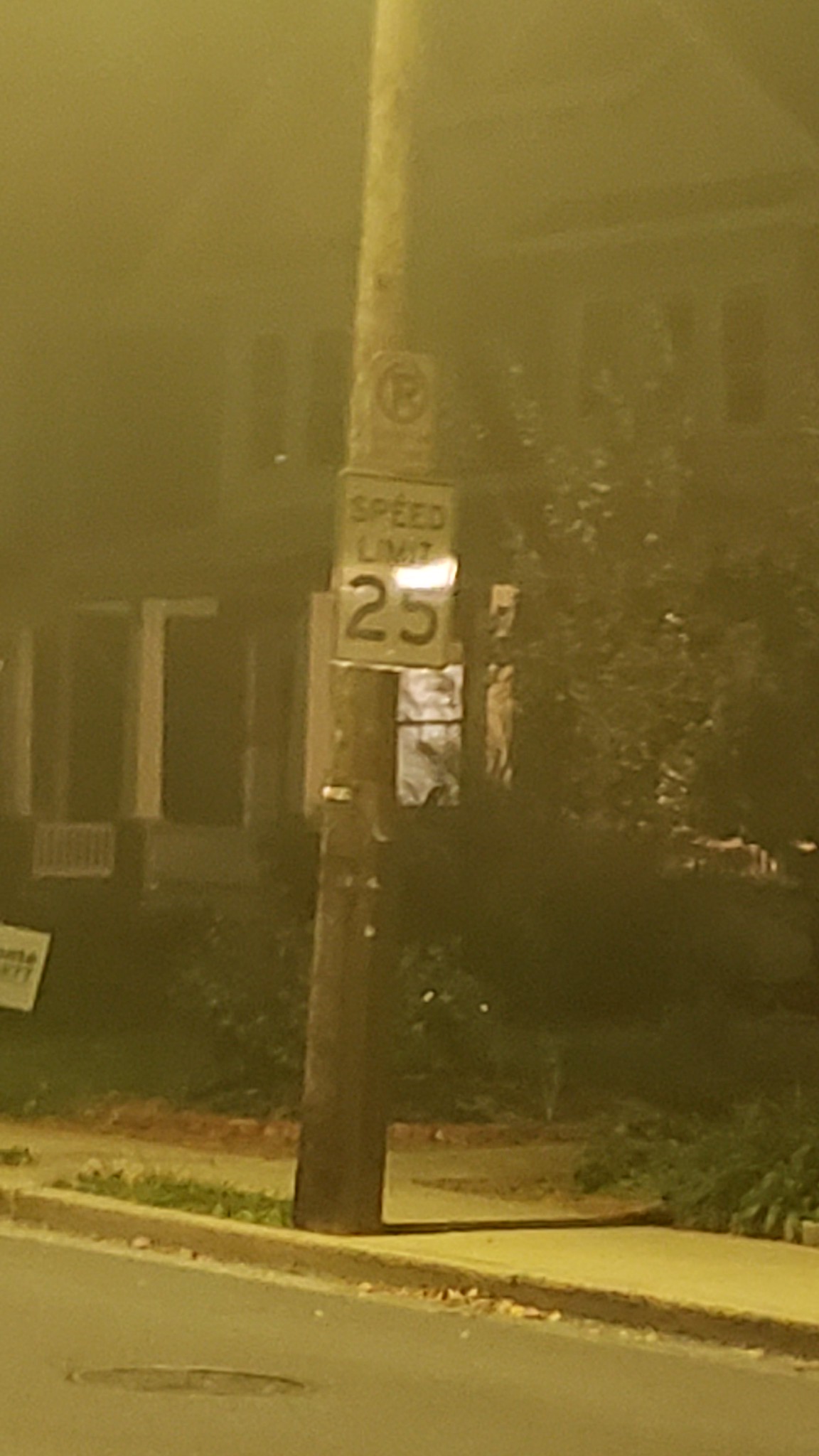A nighttime photograph captures a quiet street scene in front of a two-story house. A wooden utility pole stands prominently in the foreground, adorned with two signs. The top sign is a small rectangle featuring a black letter "P" with a red circle and a diagonal line, indicating a no parking zone. Directly beneath it, a white rectangular sign displays "Speed Limit 25" in bold black text. The house, partially obscured by the utility pole, adds a backdrop of suburban tranquility to the dimly lit scene.